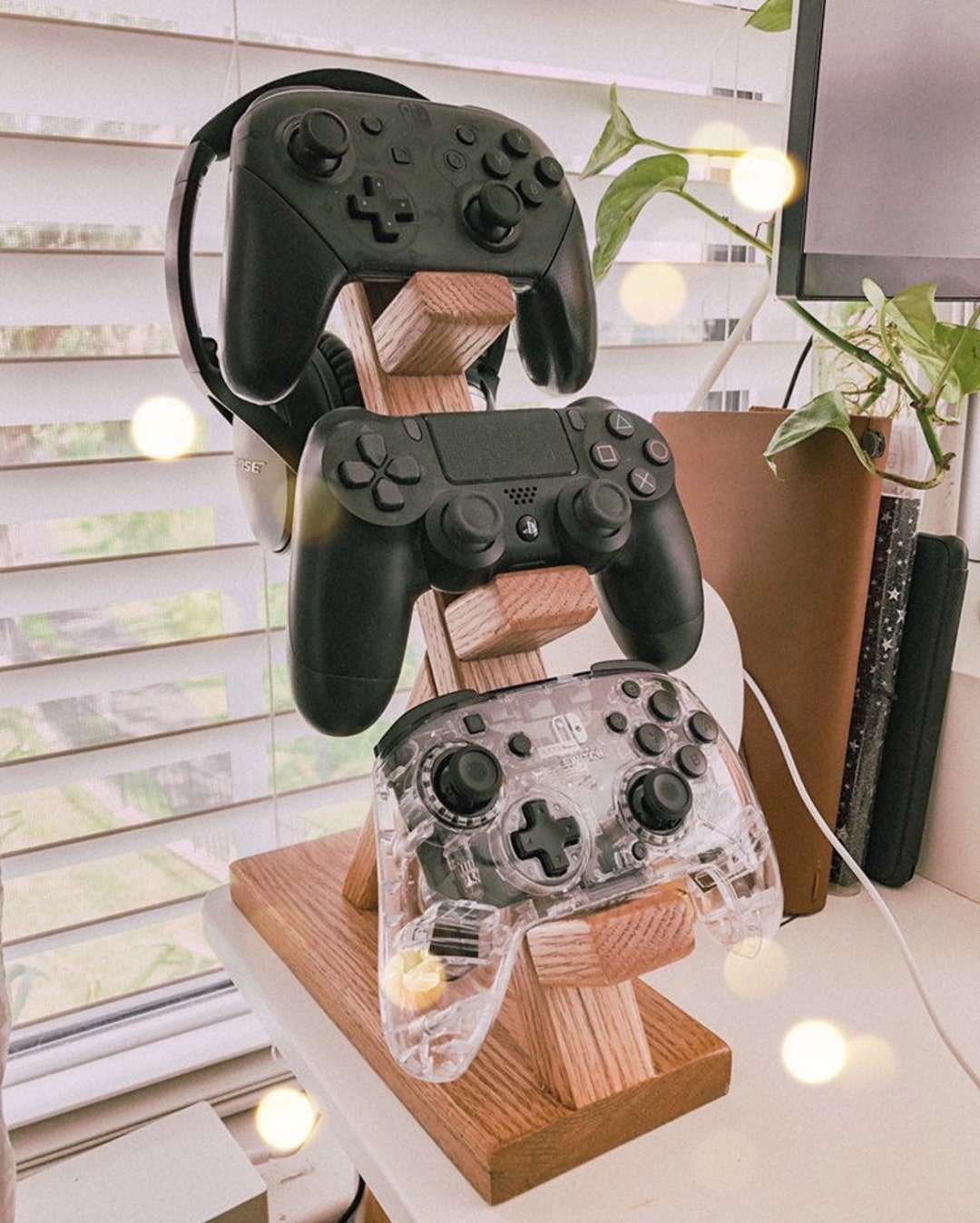In the photograph, a neatly organized display showcases three video game controllers meticulously arranged on a custom-crafted, vertical wooden stand with protruding beams that hold each controller. At the top resides a black Nintendo Switch controller, and directly below it, a black PlayStation 4 controller. The bottom position is occupied by a distinctive, transparent Nintendo Switch controller with black buttons. Above the top controller, a pair of earphones is elegantly draped. This setup is placed on a white desk, which also holds a stack of books or diaries to its right. In the background, there's a glass window with open curtains allowing sunlight to stream in, illuminating the scene. The room features some small decorative lights, adding a cozy ambiance, while greenery and trees can be glimpsed outside, indicating it is daytime. Additionally, a flat-screen display, which could be a computer monitor or a TV, is situated nearby, enhancing the gaming environment.